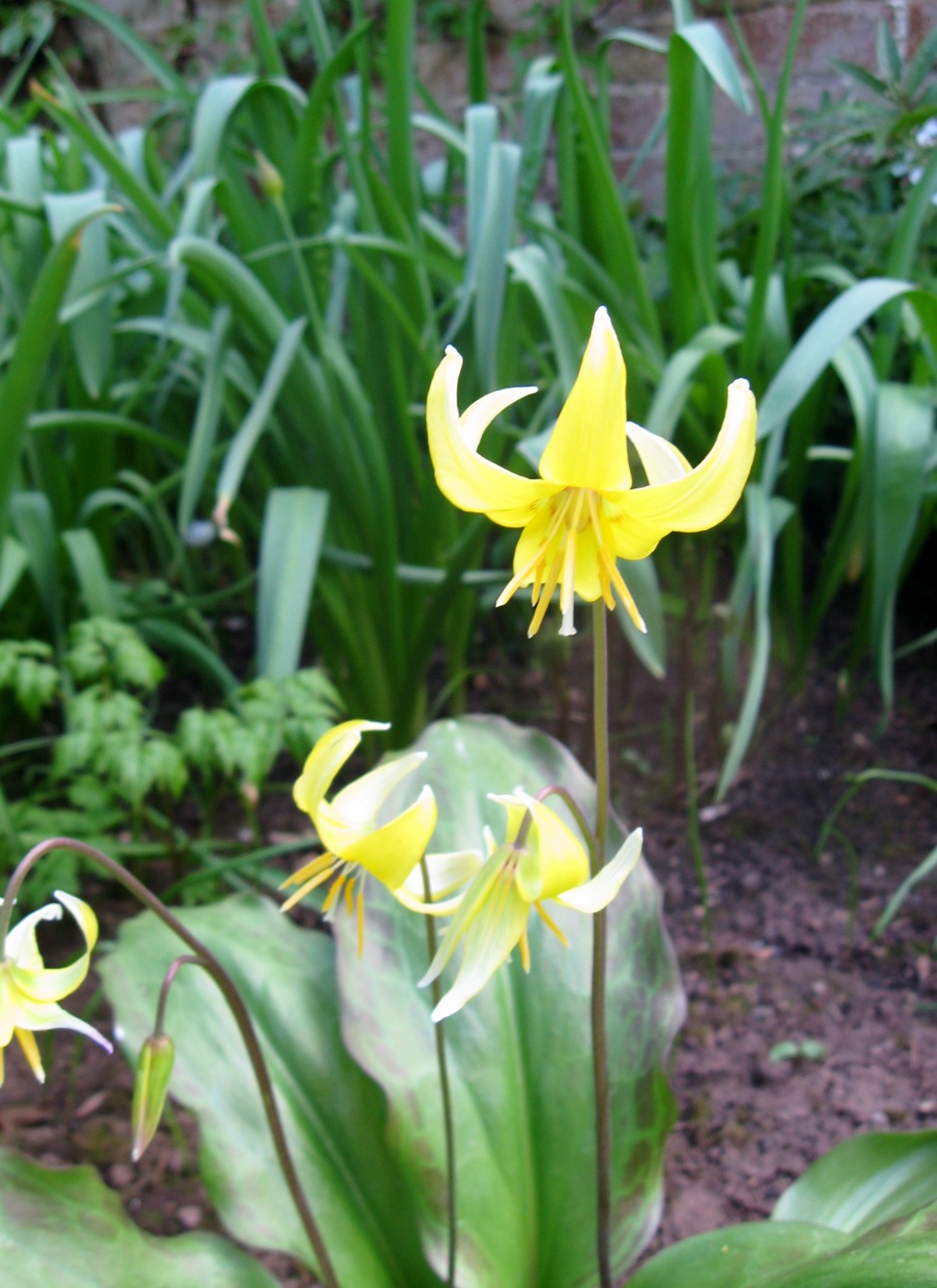This photograph captures a close-up of three graceful, yellow lily-type flowers that command the foreground of a modest garden scene. The yellow petals of these flowers face downward, resembling witch hats or orange peels in shape. They are adorned with narrow, greenish-purplish stems, extending upwards to the height of the surrounding grass. Behind these blooms, a sea of large green leaves and assorted foliage occupies the background, accompanied by visible patches of soil that suggest rows, indicative of a farming garden. The scene is bathed in soft daytime light, likely under a cloudy sky, enhancing the lush greenery and muted tones of the soil. The image, framed in dimensions reminiscent of a magazine, offers a serene glimpse into a verdant garden thriving without human presence.